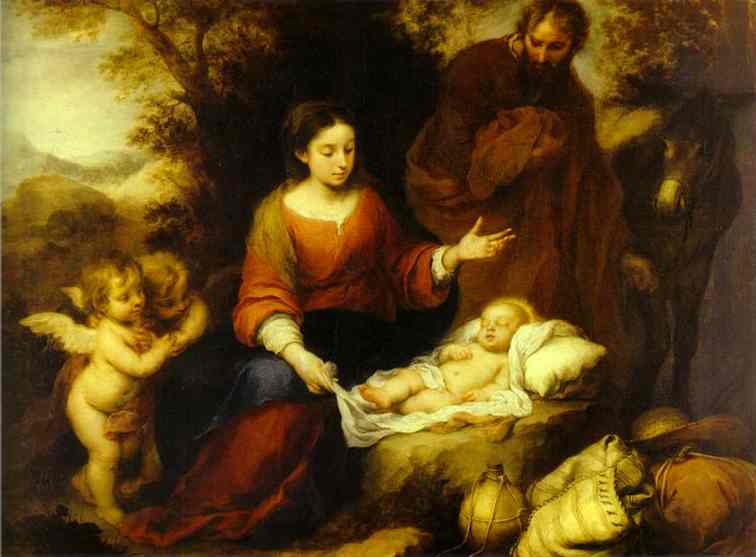This Renaissance-style painting, likely depicting a biblical scene, showcases Mary, Joseph, and the infant Jesus in a serene, forested setting. Mary is seated at the center, draped in a red dress and a blue accent, with a gold shawl around her neck. Her dark hair cascades naturally. Before her lies the baby Jesus, nestled on a rock with a white sheet and a makeshift pillow, a golden halo encircling his head. To her left, two cherubic angels observe the scene with innocent curiosity, their wings delicately spread. 

Joseph stands to the right, clad in a red or brown robe and holding part of it under his arm. He is accompanied by a donkey, indicating their journey. In the lower right, a collection of supplies, including a water bottle, suggests a brief respite amidst their travels. The background features distant, idyllic landscapes, enhancing the tranquility and depth of this heartfelt moment.